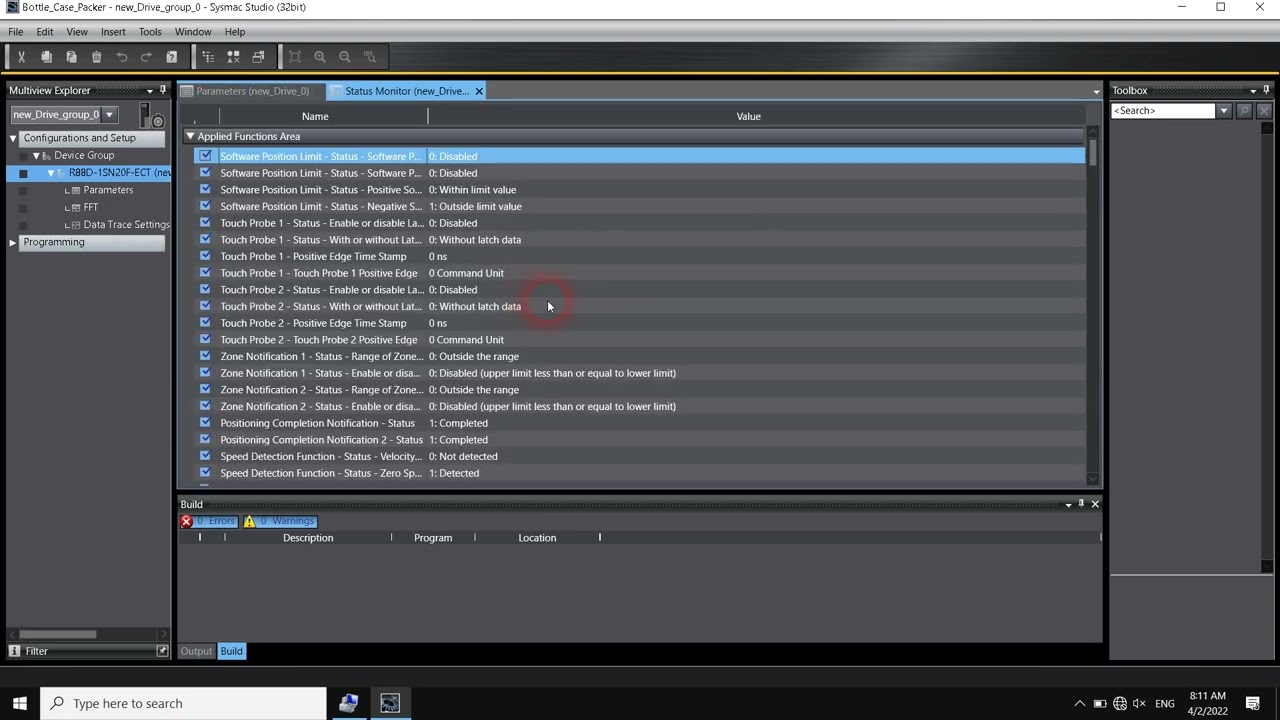This image is a screenshot from a Windows computer screen displaying a dark-themed application, possibly named Sysmax Studio. The interface appears in dark mode, with a base layer of black and white font throughout. At the top, there is a gray banner featuring the usual headings like File, Edit, and View, followed by a black toolbar with various symbols. The center of the image prominently displays a separate tab akin to what you might find in a spreadsheet or business-oriented chart, containing numerous columns of information. This tab is seemingly opened within the main application window that shows a behind layer. On the left side of the screen, there is a nested list with items labeled with terms such as "touch probe one," "zone notification one," and "speed detection function." At the bottom of the screen, the Windows taskbar is visible, including a white search bar on the bottom left and icons for Wi-Fi connection, battery status, and sound on the bottom right. The overall complexity and structure suggest it may be some kind of programming or inventory management software, but the exact purpose remains unclear.